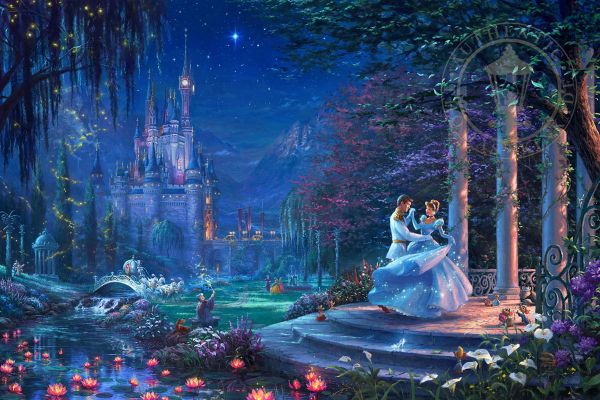In this vividly detailed scene from Disney’s animated movie "Cinderella," we see Cinderella gracefully dancing with the prince on a circular stone patio adorned with three steps, stone columns, and fireflies twinkling in the trees. Cinderella wears her iconic blue, lacy dress, her hair elegantly pulled up, while the prince is resplendent in a white jacket with gold detailing, including a belt and shoulder epaulettes. In the enchanting background, a tall, stone castle with purple and yellow highlights towers on the left. Its clock tower and steeples stand majestically under a dark blue sky peppered with tiny white stars, among which a singular blue star shines more brilliantly. A picturesque landscape surrounds them, featuring green grass fields dotted with lily pads in hues of yellow and pink. On the lawn, characters from the tale, including Cinderella’s fairy godmother holding a wand, add to the magical ambiance. A river runs along the right-hand side, crossed by a bridge, with a horse-drawn carriage in the shape of a pumpkin waiting nearby. A gazebo stands in the distant backdrop, completing this enchanting fairy tale setting.